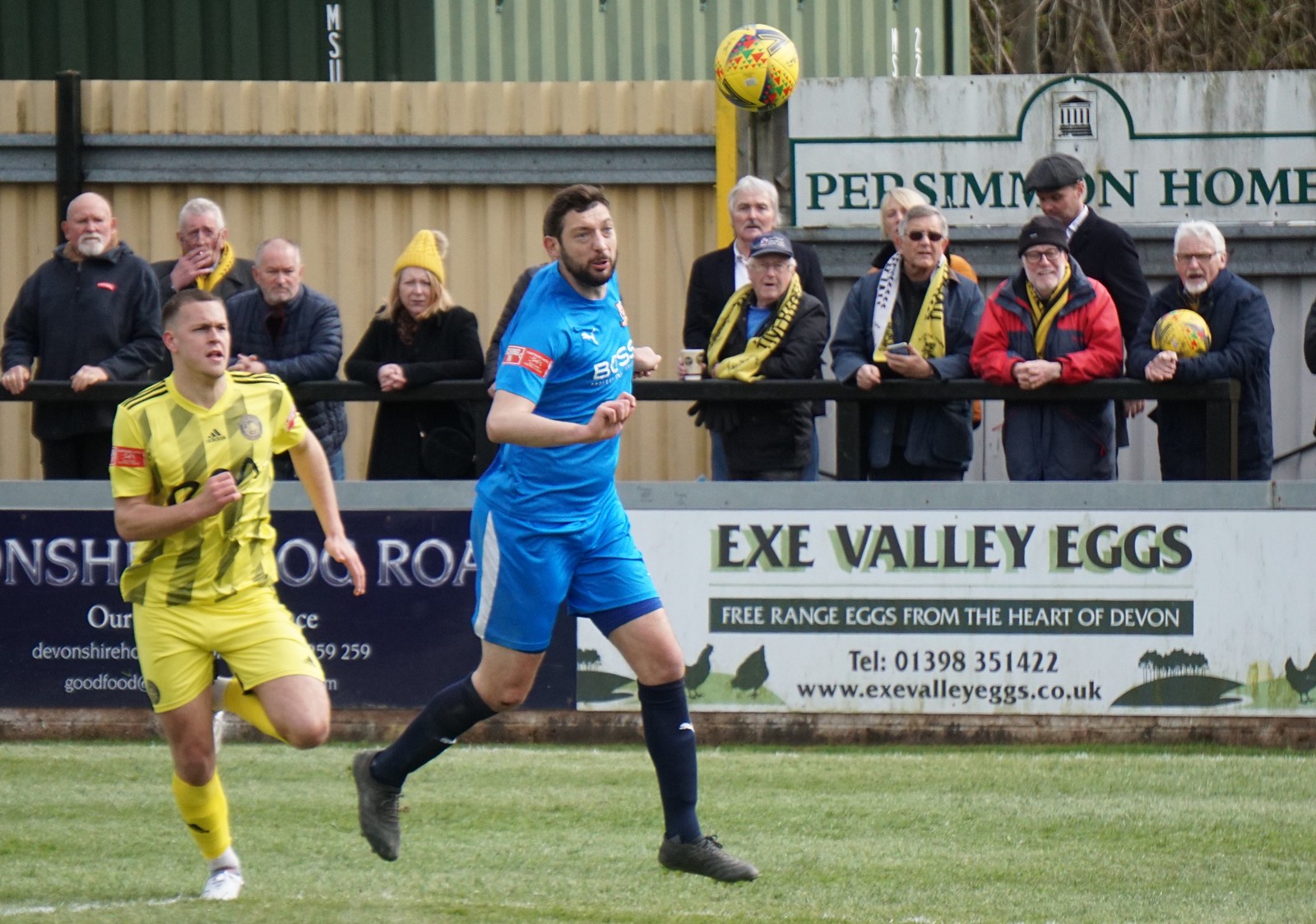The image captures an intense moment during an outdoor soccer match on a green turf field. In the foreground, two players are contending for a predominantly yellow soccer ball with red and black details, suspended mid-air at the top center of the image. The player on the left, a Caucasian with short brown hair, is wearing a yellow jersey with black vertical stripes, yellow shorts, yellow knee-high socks, and white cleats. His left leg is poised in the air, ready for action, and his right hand is clenched in a fist. He sports a red armband on his right arm. Next to him, another player, also Caucasian with a beard and short dark hair, is donning a deep blue jersey and shorts, navy knee-high socks, and black cleats.

In the background, a green banner advertising "EXE Valley Eggs" stretches behind the players, promoting free-range eggs from the heart of Devon, complete with a telephone number and a website. To the left of this advertisement is a darker banner with white lettering, partly obscured by the players. Spectators, clad in dark warm clothing and mostly male, are gathered behind a railing, indicating cooler weather. They are engaged, some with official lanyards around their necks, suggesting they might be officials or special guests. Adding to the scene, a white marble sign for "Persimmon Home" is visible behind them, situated next to a rustic brown fence, framing the lively area of spectators and advertisements.